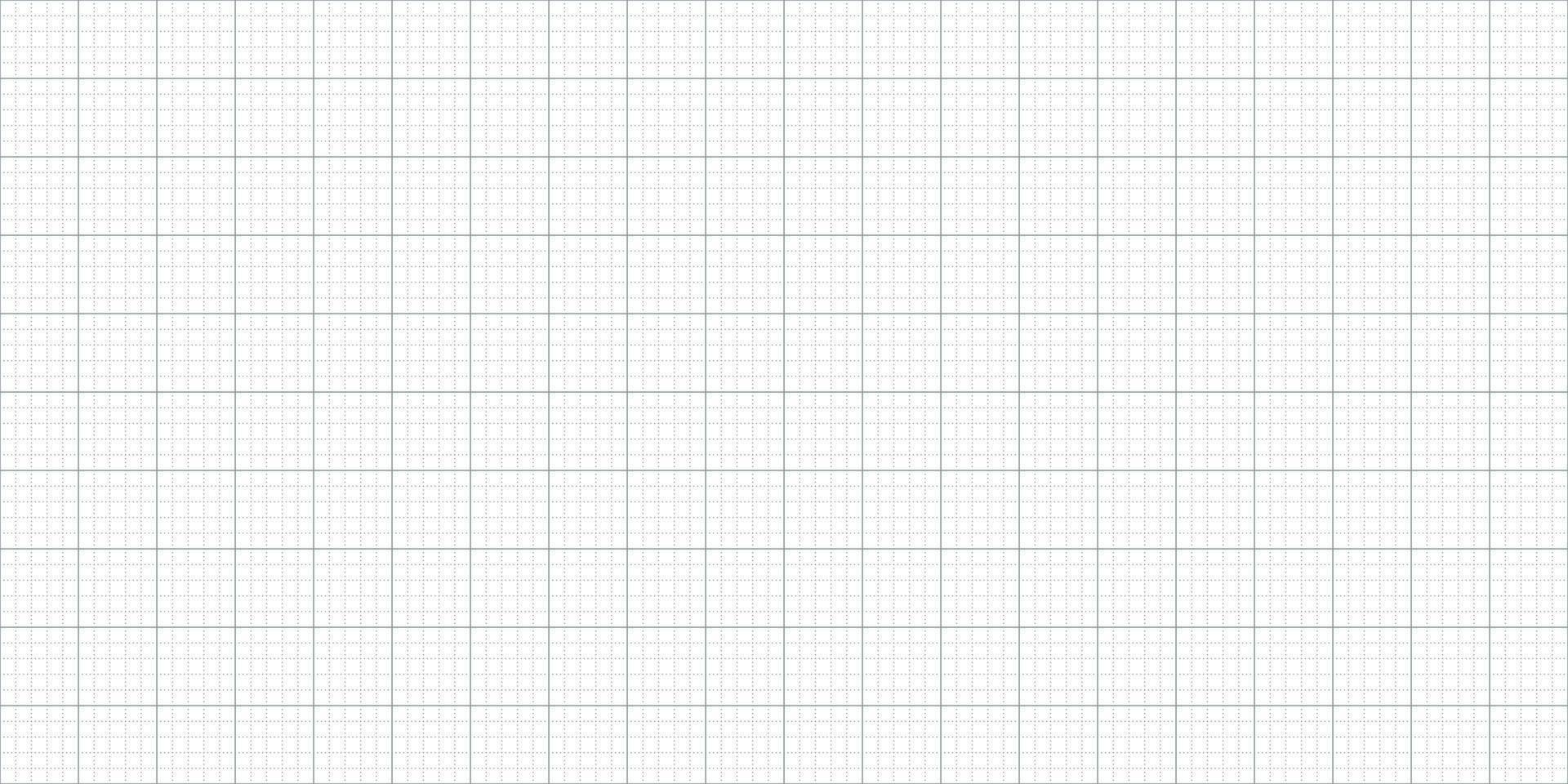The image depicts a black and white document resembling a spreadsheet or graph paper, presented in landscape orientation, wider than it is tall. It features an intricately detailed grid composed of squares. The primary grid is formed by the intersection of horizontal and vertical lines, with every fifth line being thicker and bolder in black, while the lines in between are thinner, gray, and dotted. This pattern creates larger squares, each encompassing a 5x5 array of smaller squares, totaling 25 smaller squares within each larger one. The entire grid is laid over a white background, with the smaller squares defined by thin gray lines, giving the impression of traditional graph paper used for mathematical work. The meticulous structure extends across the whole image, accentuating the detailed, structured, and repetitive nature of the grid.